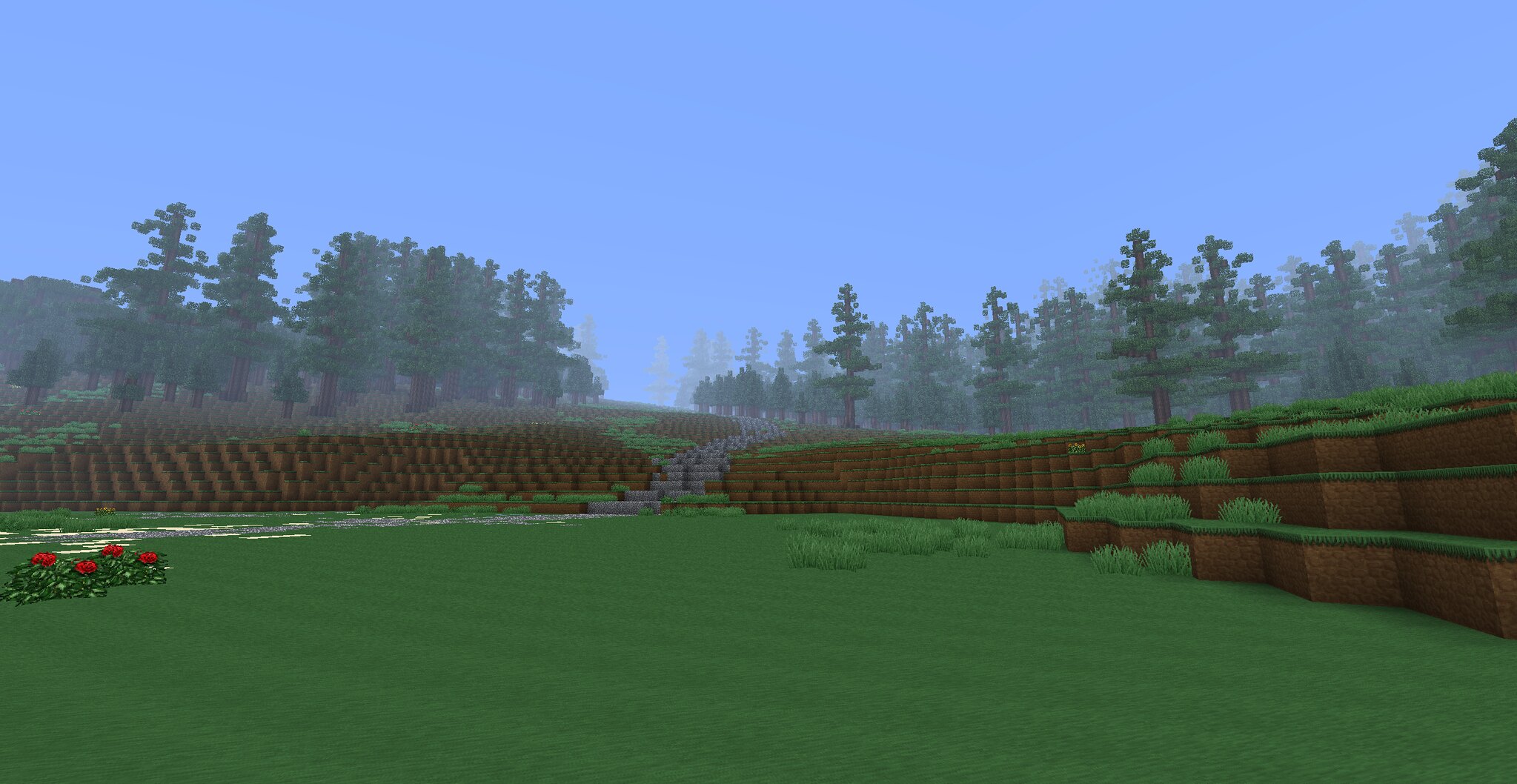A meticulously maintained field stretches out before us, showcasing lush, vibrant grass. The landscape is accentuated by rows of elegantly crafted fences made of black and brown wood; the fences are brown in the middle and black on top. Interspersed between these fences are layers of verdant plants, creating a terraced effect that draws the eye upward. Beyond the fenced layers, a dense forest of green trees rises against the horizon. Overhead, a vast expanse of clear blue sky completes the picturesque scene. A wide rock pathway meanders through the field, providing a natural pathway amidst the structured beauty. Adding a vivid splash of color, clusters of red flowers are scattered across the field, enhancing the overall charm of this serene, pastoral vista.